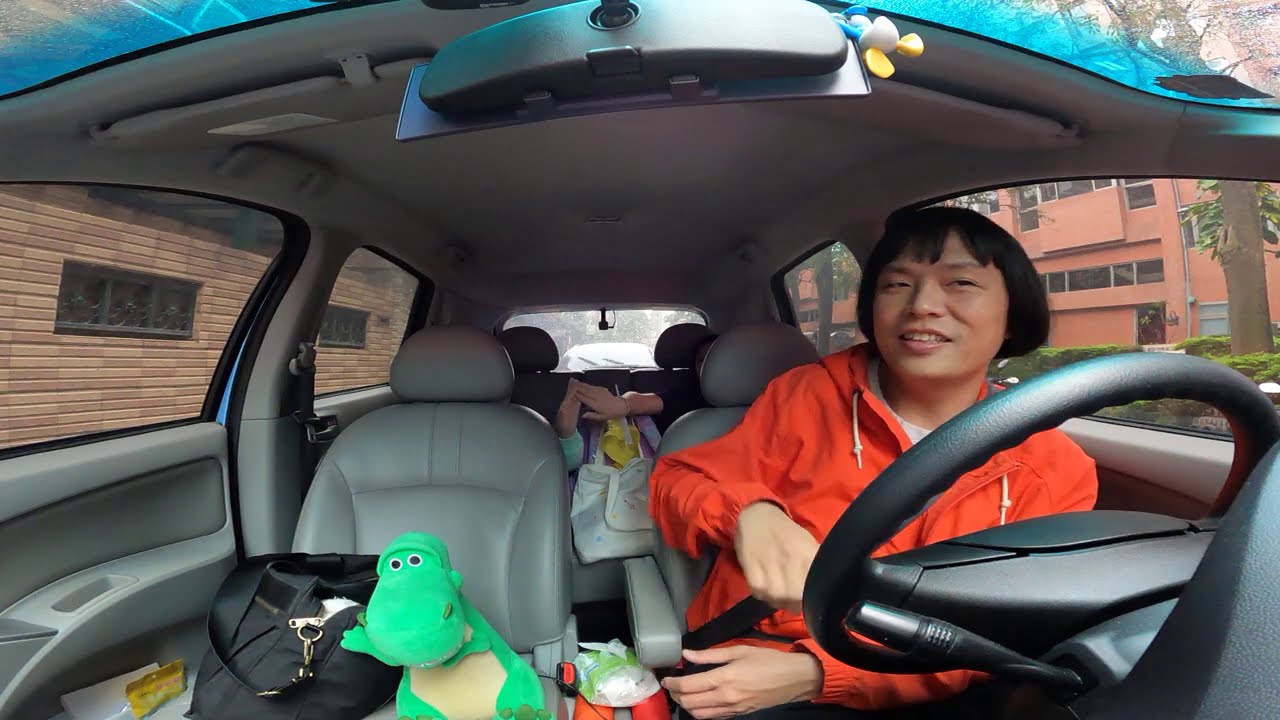Inside a well-maintained vehicle, a woman wearing an orange jacket sits in the driver’s seat with a smile on her face and her seatbelt fastened. She appears to be looking off to the side, rather than at the camera. On the passenger seat, there is a green and tan stuffed dinosaur next to a black bag. In the backseat, partially obscured by the front seats, two small hands, likely belonging to children, are touching each other as if they are performing a gentle high-five. A white bag sits between them. Outside the vehicle to the left, a brown building with multiple windows is visible, along with a few trees. Additionally, a small toy, blue with a white head and yellow ears, hangs from the rearview mirror, adding a playful touch to the scene. The image captures the interior of the vehicle in the middle of the day, with various shades of orange, green, brown, and other colors adding vibrancy to the composition.